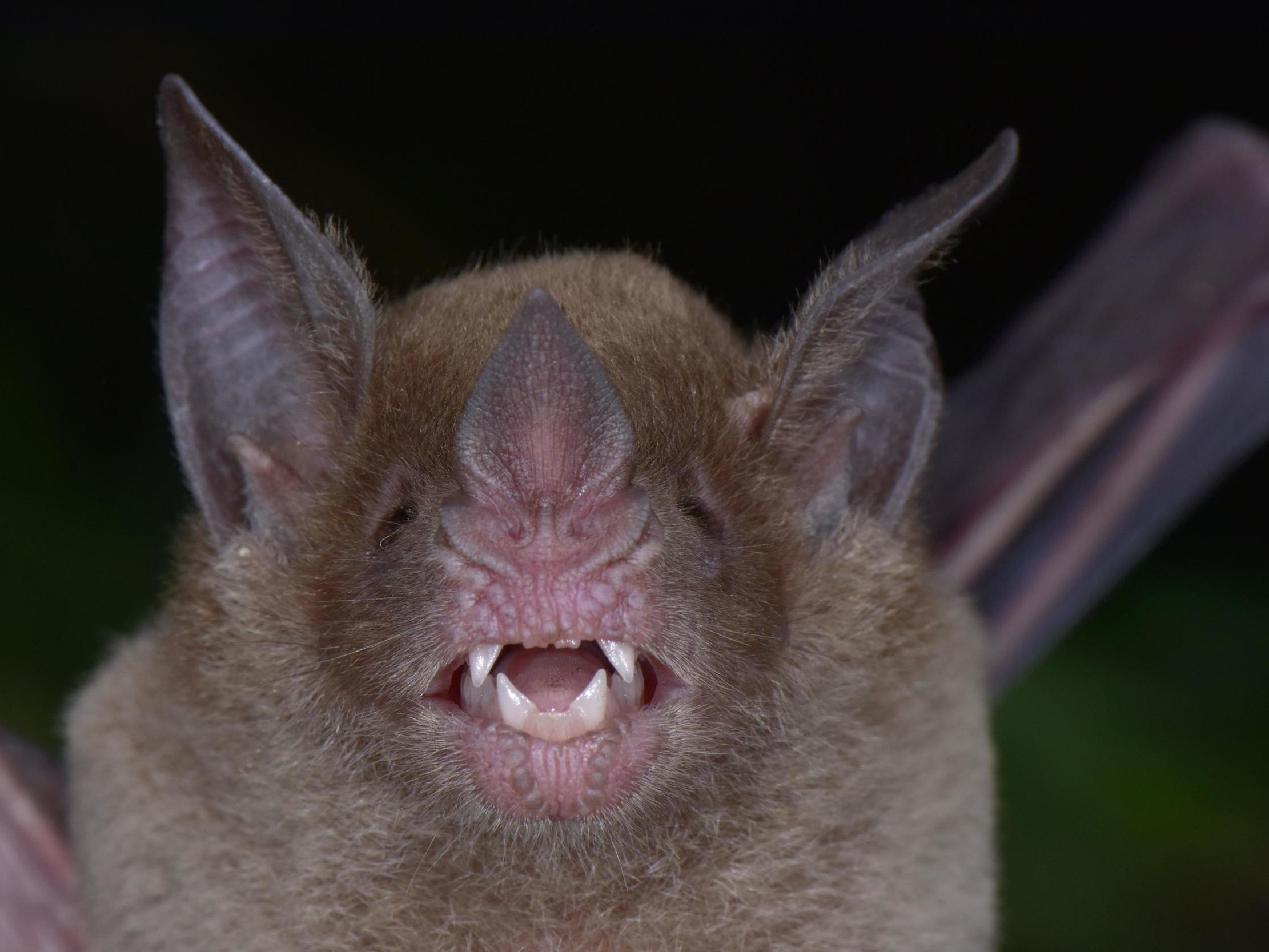This close-up photograph captures a detailed view of a bat against a blurred night-time background. The bat's face is prominently featured, displaying its open mouth with sharp white upper and lower fangs. Surrounding the bat's mouth is pink flesh, with its nose—which has a diamond or triangle shape—showing a pink underside and a dark brown top. Its black eyes are slightly less conspicuous due to the structure of its face. The bat's ears are large, pointy, and covered in thin, dark fur with lines running through them, showing a mostly dark pink and black interior with a few spare hairs. The bat's head fur is a rich chocolate brown that lightens towards its nose. This lighter brown fur extends down its torso. The right wing of the bat is partly visible and appears dark black or brown, with its interior showing a blurred pinkish hue. The left wing is cut off in the photograph. Overall, the image illustrates the intricate features of this nocturnal creature, framed by a predominantly dark and slightly green-tinged background.